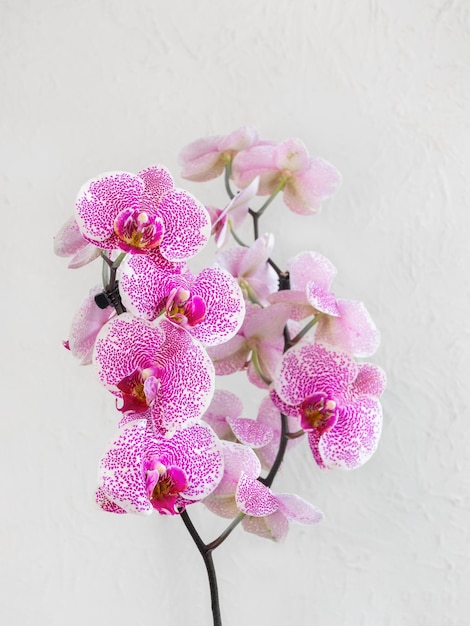This close-up image captures a cluster of stunning orchids set against an off-white background. The composition is taller than it is wide, creating a vertical frame that highlights the elegant stems of the flowers. The orchids, predominantly bright purple with whitish and pinkish petals adorned with dark pink dots, feature prominently. There are approximately five blossoms in full bloom facing the camera, with four on one stem and one on an adjacent stem with several other blooms emerging in various directions. The petals are oval-shaped and smooth, with some displaying a mesmerizing swirl of pink hues. The darker centers of the flowers contain whitish-yellow bulb-like structures, giving way to subtle green accents. The stems, a deep dark green with possible hints of brown, contrast beautifully with the vibrant petals. This image, whether a photorealistic painting or a computer-generated rendition, presents a botanical marvel, likely orchids, in exquisite detail.